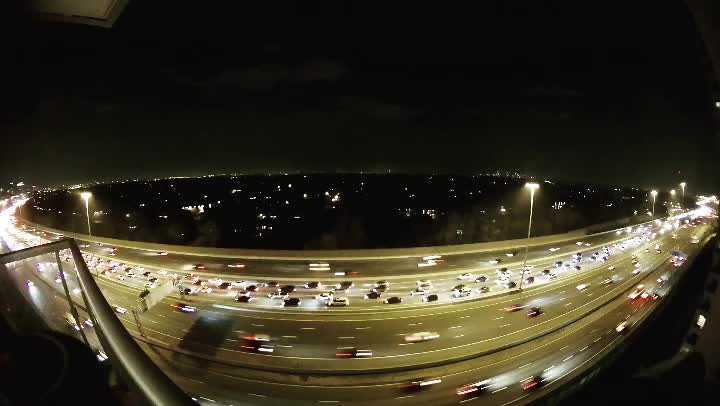This vibrant color photograph, captured from an elevated vantage point, showcases a bustling freeway at night. The scene is composed with numerous lanes filled with vehicles. In the foreground, the cars appear as streaks of light, indicating their swift movement. In contrast, the background reveals a stark difference; traffic is heavily congested with stationary cars. The image was shot with a fisheye lens, which adds a dramatic curve to the road, enhancing the sense of dynamic motion. The night sky is an inky black, devoid of stars, casting a stark contrast to the streetlights that dot the scene and illuminate the road below. City lights twinkle faintly in the distance. The photograph is distinctly wider than it is tall, capturing the vast expanse of the freeway. The absence of visible people in the image directs full attention to the relentless flow of traffic and the urban landscape, emphasizing the city's ceaseless activity.